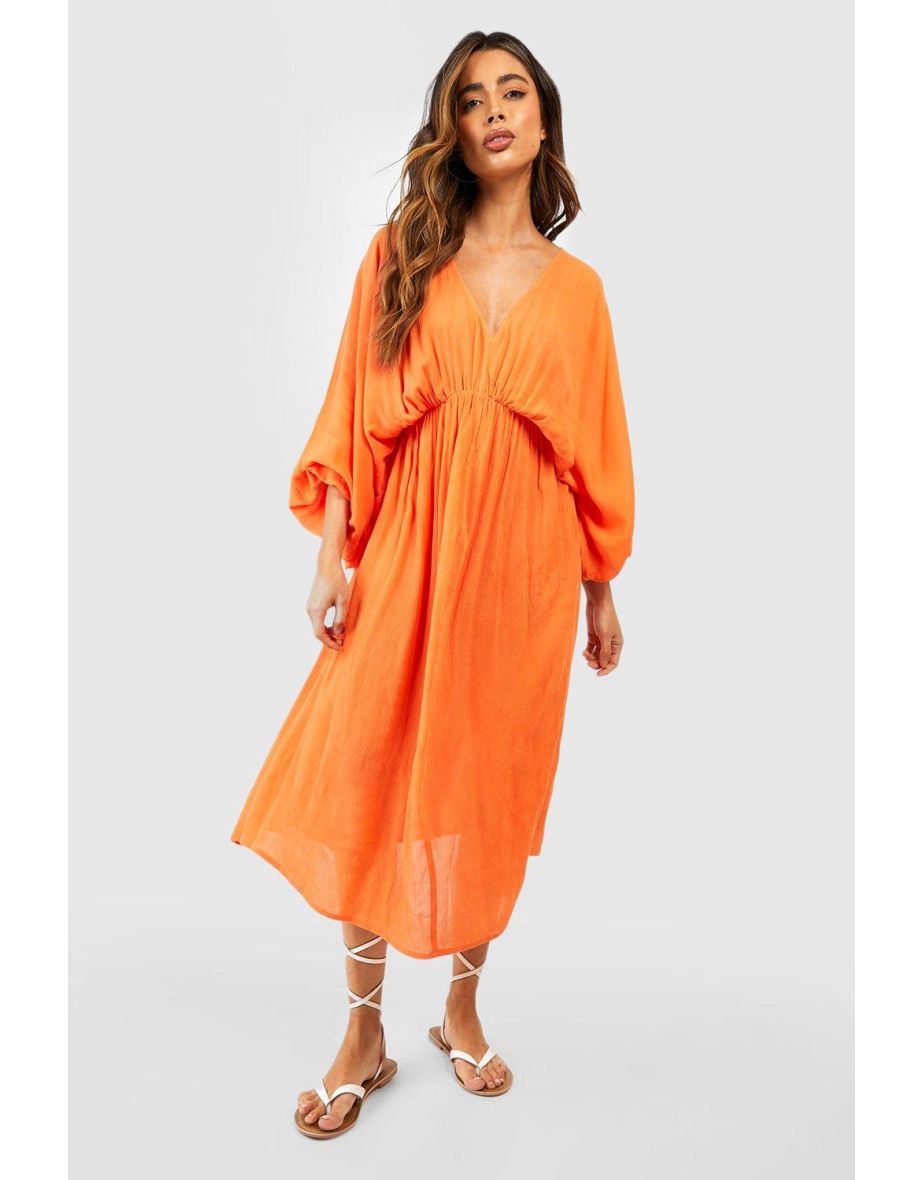This photograph features a woman with long, wavy brown hair that flows down to her chest, adorned with lighter brown or blonde highlights. Her hair is elegantly styled, with one side cascading over her shoulder and the other falling down her back. She is dressed in a striking orange dress that cinches just under the bust, giving it a ruched, drawstring effect. The dress has a loose, slightly baggy fit around the arms and chest, with sleeves that gather at the wrists, creating a relaxed, draped look. The dress extends to her calves and appears slightly see-through towards the bottom, although it is lined to prevent any opacity issues.

The woman exudes confidence with a somewhat condescending expression, looking down at the viewer. Her makeup is flawless, highlighting her lips and adding to her overall put-together appearance. She has a tan complexion, contributing to a potential holiday vibe for the outfit.

Completing her ensemble, she wears white gladiator-style sandals with straps that cross along her legs. The background of the image is a simple, solid gray, ensuring that the focus remains entirely on her stylish presentation.